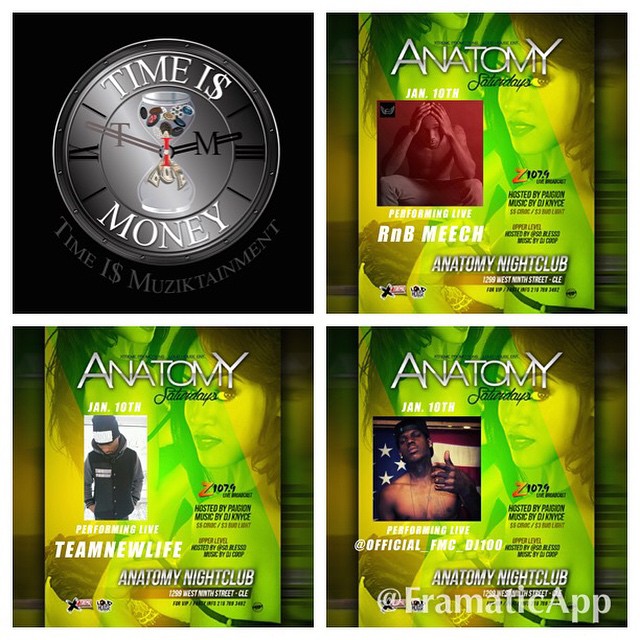The image features a 2x2 grid of four distinct flyers. The top-left flyer has a prominent round gray-silver clock on a black background, with the phrase "Time is Money" printed inside in white. Underneath, it states "Time is Musictainment." The remaining three flyers are similarly themed, promoting "Anatomy Saturdays" at the "Anatomy Nightclub," located at "1299 West 9th Street." The top-right flyer is bright yellow and green, featuring two women in the background and detailing an event on January 10th. It highlights performances by different artists across each flyer: the top-right shows a photo of a black male, "Performing Live R&B Meech," supported by Z1074 and Pagan Music by DJ Nice. The flyer on the bottom-left follows the same design but highlights a different black male artist, "Performing Live Team New Life," while the bottom-right flyer, also identical in layout, features yet another black male artist, "Performing Live Official FMC D1100." The visuals of each performing artist differ: the top-right male holds his head in a red atmosphere, the bottom-left male is looking down with a hat adorned with a white spot, and the bottom-right male appears shirtless, making a gun gesture with an American flag backdrop.